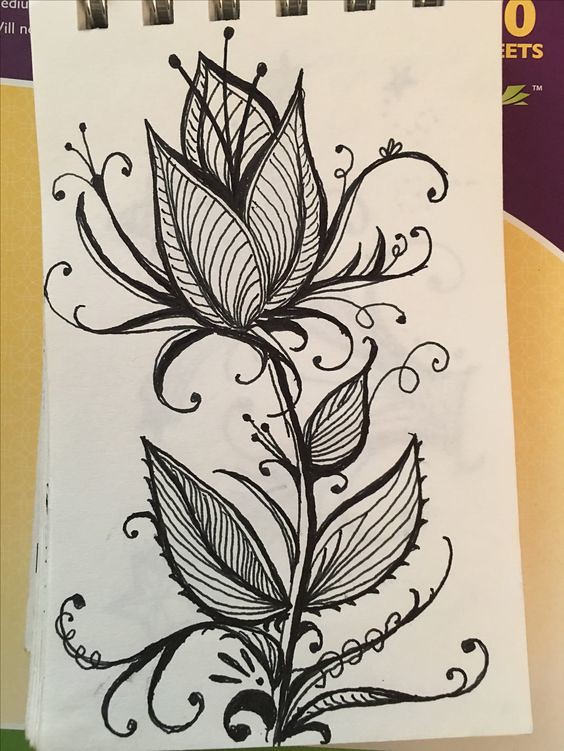This image captures a sketchbook open to a white, slightly yellowish page featuring a meticulously detailed pen drawing of a tulip-like flower. The sketch is rendered in black ink, with darker areas providing shading. The flower has three prominent antenna-like structures extending from the bloom, and its stem is adorned with three leaves. The base of the plant includes circular, curled foliage. The sketchbook's metal binding rings are visible at the top, suggesting the page is part of a spiral-bound notebook. This notebook lies against another with a distinct yellow cover, adorned with a purple stripe curving down from the top. Between the yellow and purple sections, there's a narrow white stripe. Visible text includes parts of the phrase "zero eats" and possibly "medium" in white lettering.